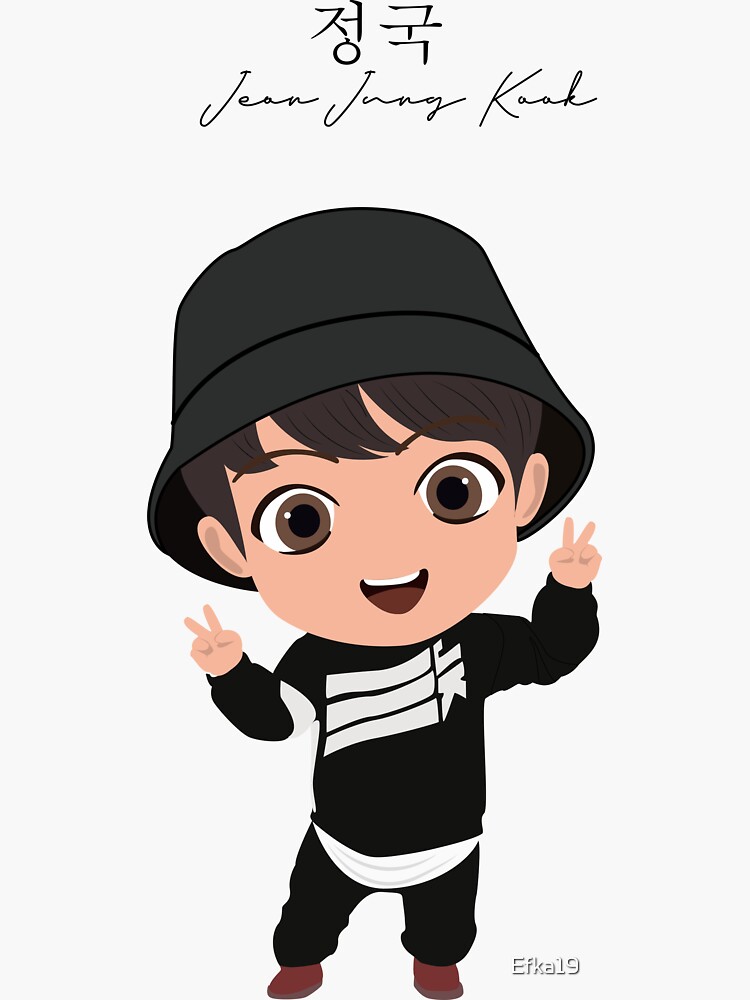This vertical rectangular image features a cartoon figure of a young boy, possibly inspired by a Japanese cartoon style. He has large brown eyes, a big smile showing his top teeth, and a lot of dark hair peeking out from underneath a black bucket hat. The boy is dressed in black sweatpants and a black crewneck sweater with white lines across it and the initials "JK" prominently displayed on the right side. Peeking out from underneath the sweater is a white t-shirt that hangs untucked over his pants. He is striking a playful pose with both arms raised and fingers making the peace sign. His ensemble is completed with brown shoes. The image also includes artistic details such as shadowing in his ears. At the top of the image, there is a signature that appears to read "Jin Jung Kook" along with two Japanese characters. Additionally, there is a watermark at the bottom right corner, attributed to "EFKA19."